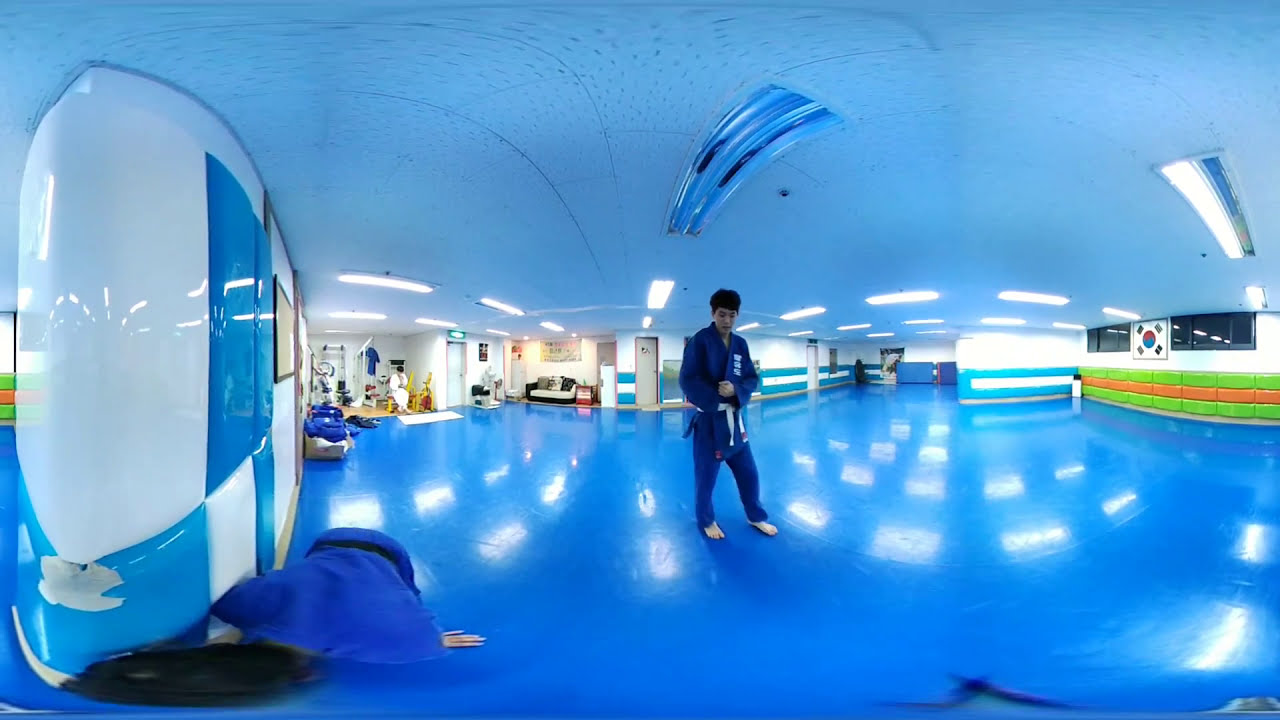The image is a 360-degree shot inside a modern martial arts studio with an overall blue tint due to the lighting. The space features a glossy, shiny blue floor that reflects long light strips from the ceiling, enhancing the room's futuristic feel. Central to the photo stands a young Asian man in traditional martial arts attire—a blue gi with a white belt tied at the front. He is barefoot, gazing downward with his arms and hands positioned in front of him. In the bottom left corner, another person with black hair is crouched on all fours, similarly dressed in a blue uniform but distinguished by a black belt, with their back facing the camera.

The background features an orderly array of equipment and seating along a white wall adorned with blue padding. To the right, there's a line of green and orange pads, contributing to the room's vibrant color scheme. On the left side, shiny plastic walls display various martial arts jackets and uniforms. An exit doorway and additional doors are visible along the back wall, which also includes a window near the ceiling and a white flag with black square markings. Despite the camera lens distortion bending the space, the photo captures the studio's unique and colorful post-modern design.